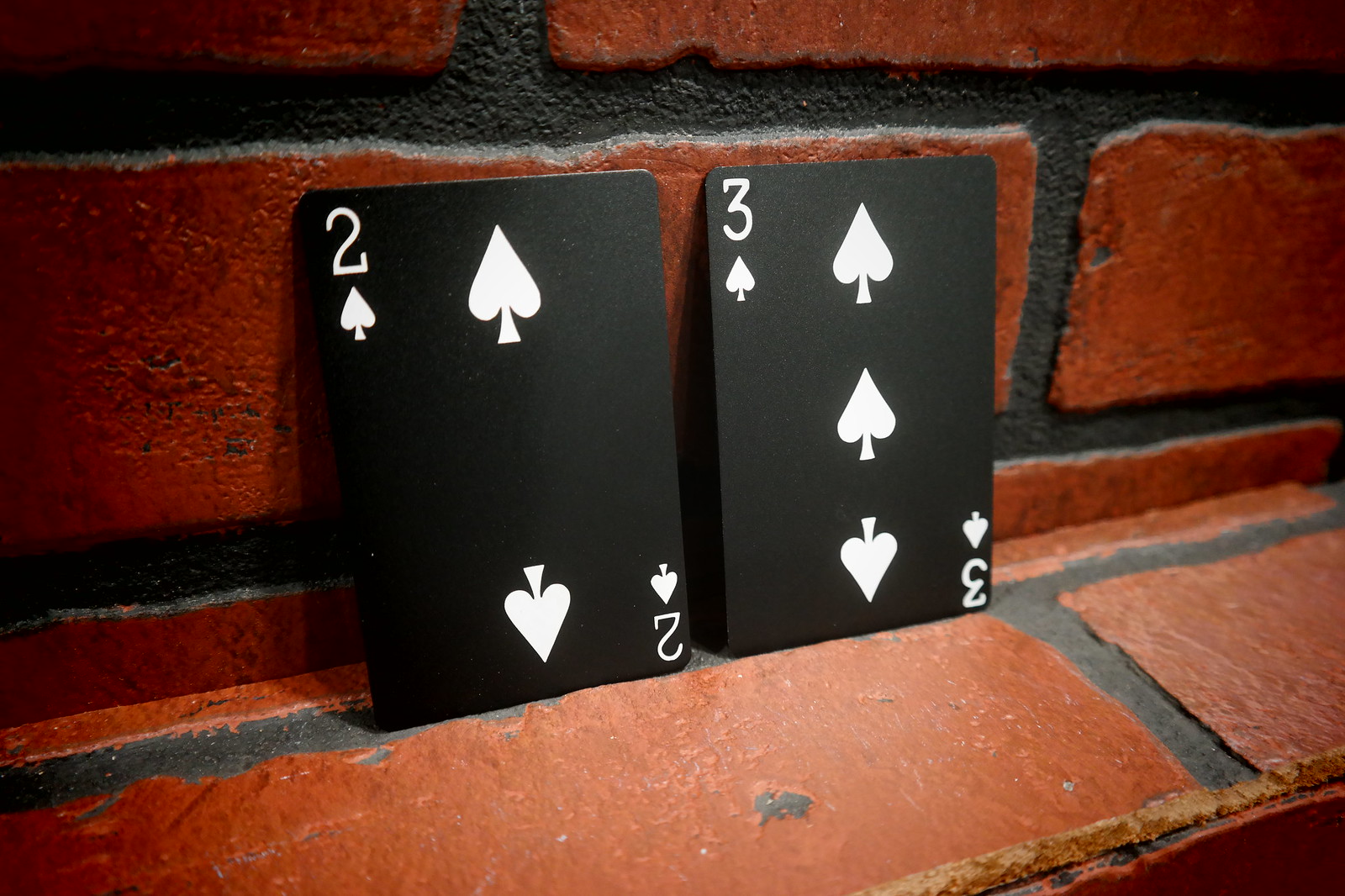This color photograph features a red brick wall with distinctive black grout outlining each brick. Directly in the center of the image, there is a ledge made of the same red bricks and black grout. Resting against this ledge are two playing cards, specifically the Two of Spades and the Three of Spades.

The Two of Spades card displays two upright spade symbols, one each in the top left and bottom right corners, with an additional two spades arranged in the middle. Similarly, the Three of Spades card to its right showcases three spade symbols and corresponding numbers. The number three is represented twice: once upright with a spade below it in the top left corner, and once upside down in the bottom right corner.

Both cards are primarily black, with the spade symbols and numbers printed in white, creating a sharp contrast. They are positioned against the brick wall, nestled neatly in the crevice where the grout forms a vertical line. The lighting accentuates the textures of the brick and the ledge, highlighting the stark black-and-white imagery of the playing cards.